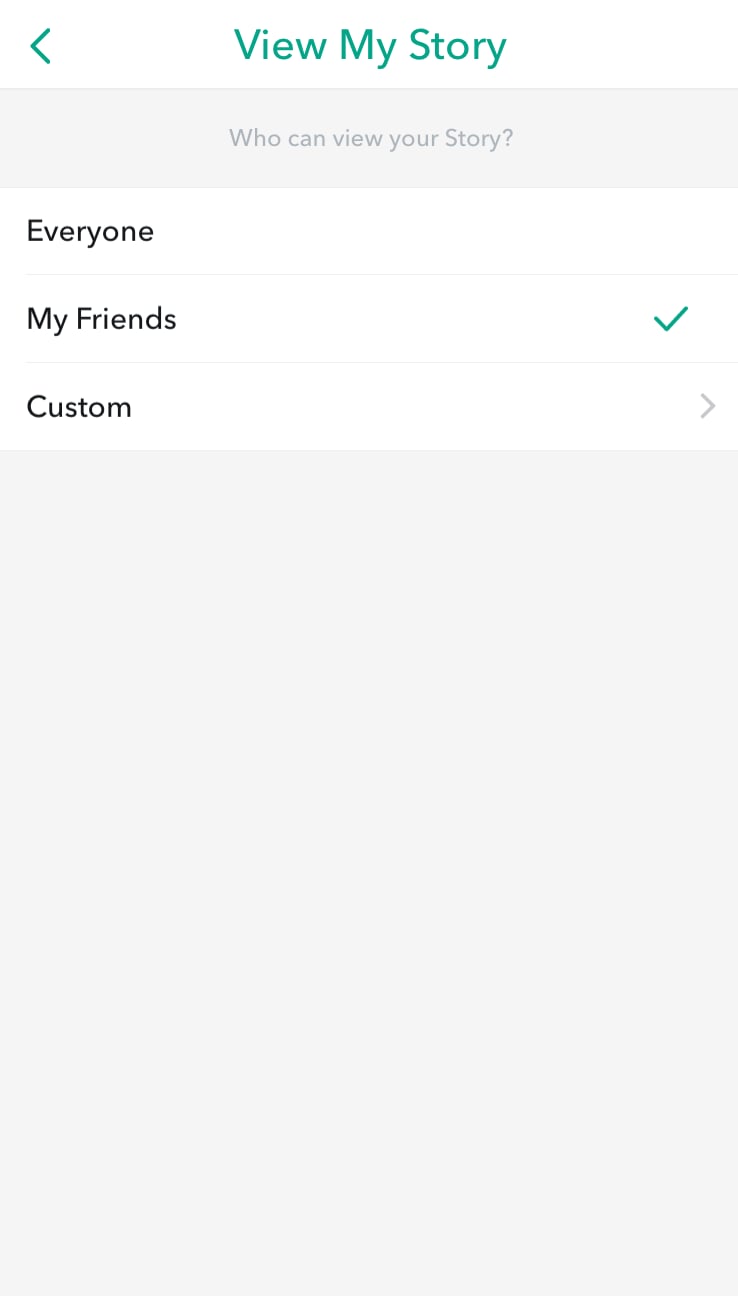This image is a screenshot from a mobile app, displayed in portrait orientation akin to a cellphone screen. The top section features a white background with a green left arrow icon and centered green text that reads "View My Story." Below this, there is a long rectangular gray box with the text "Who can view my story" in gray font. 

The interface is divided by thin gray lines into distinct categories and selectable options. Three horizontally-aligned boxes are present: "Everyone," "My Friends," and "Custom" (which has a right caret indicating further options). The "My Friends" box is checked with a green check mark, suggesting it is the selected option.

Further down, there's another long, gray rectangular box filled with blank space, slightly taller than it is wide. This layout indicates that the user is on a page within the app where they can decide the visibility of their story posts, opting to share them exclusively with their friends rather than a wider audience.